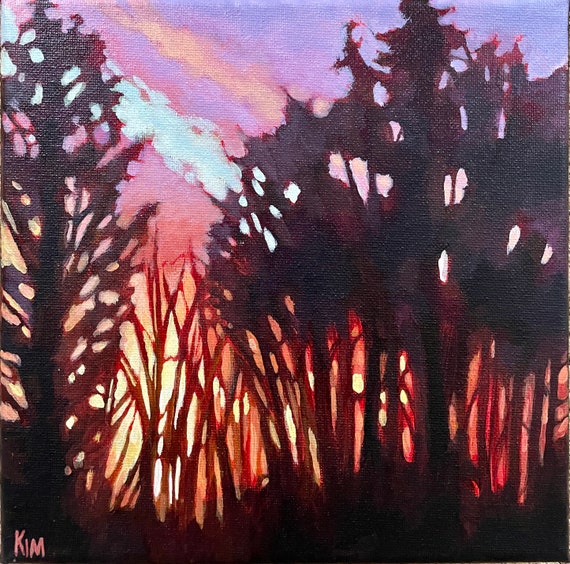The painting depicts a woodland area seemingly engulfed in a forest fire, showcased with photorealistic detail and a slight blur. In the foreground, dark, silhouetted trees and high grasses stand out against the illuminated backdrop. The left side features a towering pine or fir tree, and further right, narrow tree trunks rise into billowing leafy tops. The center of the image is dominated by smaller bushes, bathed in a glowing orange light that hints at a fire, although no flames are visible. The sky above is a mix of pastel hues—pink, purple, and light blue—interspersed with horizontal wisps of clouds, reflecting the fiery sunset glow below. At the top right, the sky darkens into a pure black silhouette of trees. The ground is shadowed, yet pierced by rays of light, enhancing the dramatic effect of the scene. Notably, the bottom left corner of the canvas bears the signature "Kim" in pink lettering, grounding the composition with a personal touch.